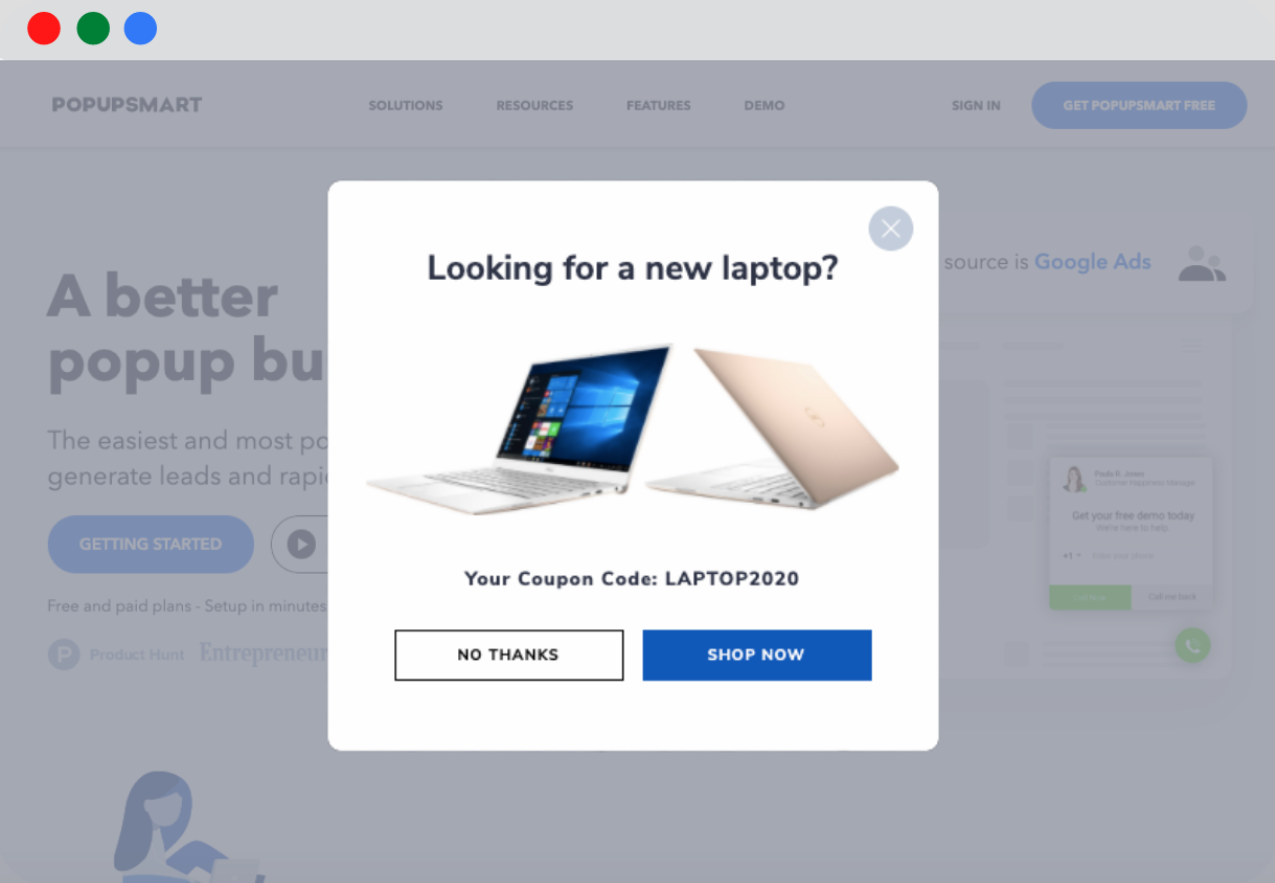The image is a horizontal screenshot captured from a computer screen. The top portion of the web page features a light to medium gray gradient. In the upper left corner of the browser window, three small circles are visible: the leftmost circle is red, the middle one is green, and the rightmost one is blue. Below this, the main content of the webpage is slightly grayed out due to an active pop-up box. 

In the background, the partially visible webpage header reads "Pop-up Smart," with navigation options including "Solutions," "Resources," "Features," and "Demo." Additionally, there are buttons for signing in and obtaining Pop-up Smart for free, with a prominent blue button available for interaction. Some text about getting a free demo and contacting someone is partially obscured by the pop-up.

The pop-up box itself is white and centrally located on the screen. It prominently asks, "Looking for a new laptop?" with a gray 'X' in the upper right corner for closing the pop-up. The box displays two images of laptops and offers a coupon code. At the bottom of the pop-up are two clickable buttons: "No Thanks" and a blue "Shop Now" button.